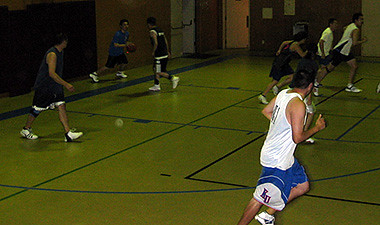This photograph captures an intense moment of a basketball game featuring six men actively engaged on the court. The players are dressed in various athletic attire: two in white tank tops, one in a white short-sleeved shirt, three in darker-colored tank tops, and one notable player in a blue t-shirt who currently has possession of the basketball. The court itself has a blond wood tone with distinct black and blue markings that segment the playing area. Situated in an indoor setting, the background includes various doors—some with wood-toned finishes and others in white—adding depth to the scene. Despite the grainy quality of the image, the details of the players' movements and outfits are clearly visible. All players are wearing shorts and sneakers, and some appear to be in mid-motion, emphasizing the dynamic nature of the game.